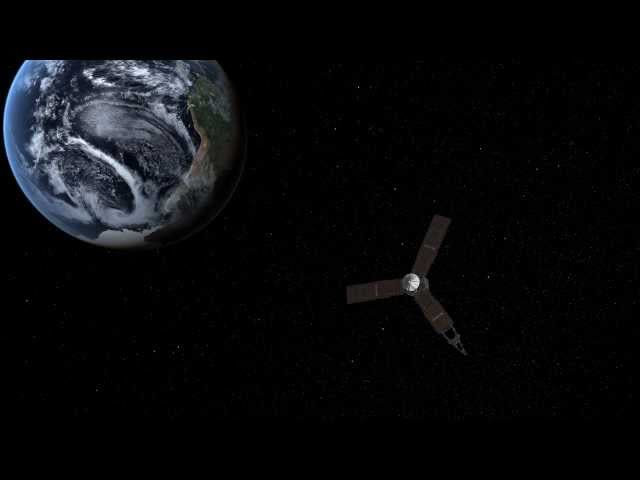This detailed computer-generated image, possibly from educational material or a video game, showcases a tranquil space scene with the Earth and a satellite in the foreground. The background is primarily black, filled with faint stars, emphasizing the vastness of space. Earth occupies the top left portion of the image, displaying vivid blue oceans, green landmasses like Africa, and swirling gray and white cloud formations, indicative of the planet's vibrant atmosphere. The globe's curvature is evident, though its top is partially cut off.

In the middle right, a detailed satellite appears, seemingly small against the backdrop of Earth. The satellite has three distinct, brownish solar panels, resembling wings, one of which features a metallic attachment possibly serving as an antenna. The central structure of the satellite includes a white cap and a prominent body, intricately designed for space exploration. The satellite seems directed away from Earth, suggesting it might have just been launched or is on a mission, its position highlighted by the large, round presence of Earth juxtaposed against the endless void of space.